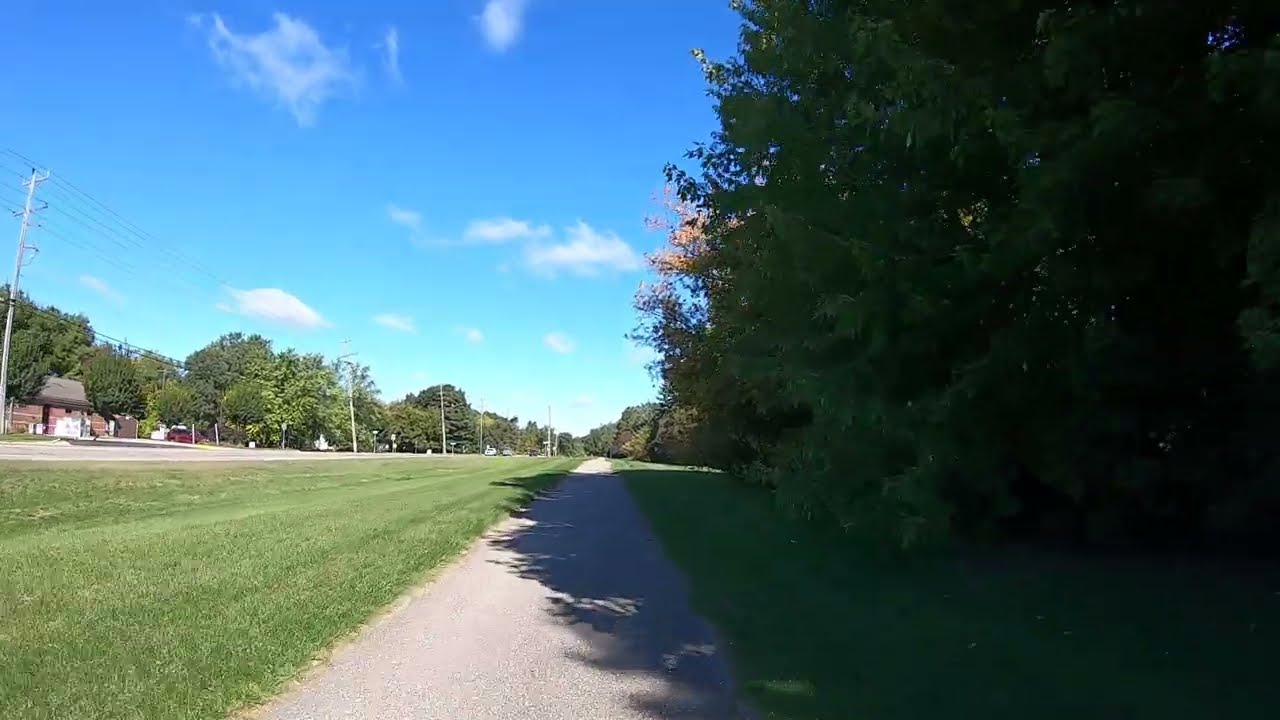The image depicts a sunlit dirt or asphalt walking trail flanked by lush green grass on both sides. On the right side of the path, a large tree provides ample shade, creating a significant shadow across the trail and allowing only specks of sunlight to filter through. In the distance, the trail continues straight, surrounded by more trees. To the left of the trail, beyond the grass, there is what appears to be a road accompanied by telephone poles and several residential buildings. A parked vehicle is visible in what seems to be a driveway near these buildings. The weather is clear with a bright blue sky dotted with a few clouds, particularly concentrated on the left side of the image. The entire scene is well-lit by natural daylight and shows no people or text. The photo is captured from about torso height, offering a clear and detailed view of this tranquil outdoor setting.